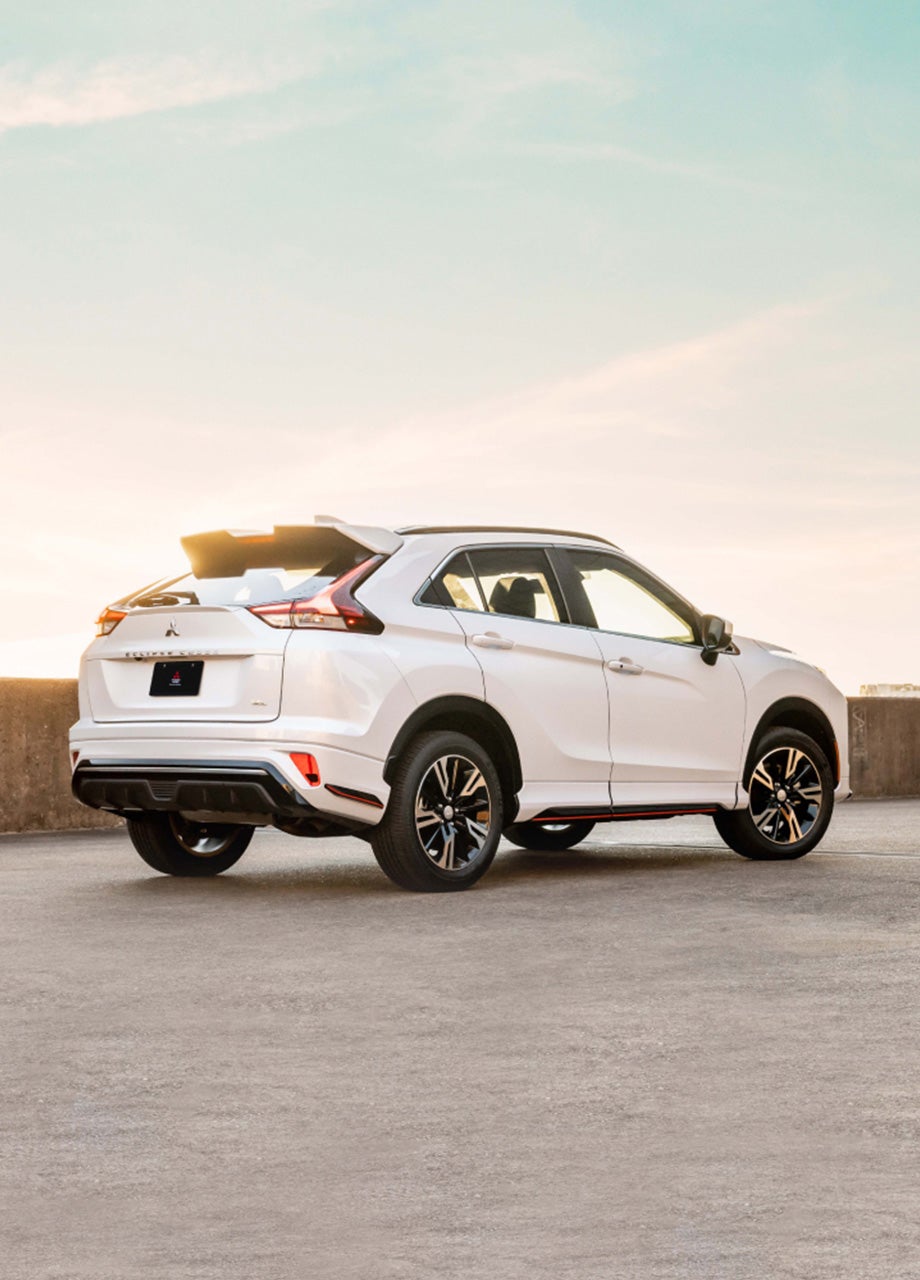The photograph features a pristine, white, four-door Mitsubishi SUV parked on a concrete or gravel platform near a scenic location, possibly by the ocean or a dam. The SUV gleams with chrome wheels and modern design, suggesting it's a recent or current model. The perspective captures the vehicle from a rear-side angle, revealing its bright rims, a visible logo, and a license plate on the back, which might also include a spoiler. The scene is bathed in sunlight, casting reflections and a gentle glow on the SUV's surface, indicative of a bright blue sky with an orange hue from the setting sun. Faint clouds dot the sky, enhancing the image's natural atmosphere. Behind the vehicle, a concrete barrier and some brown brush are visible, adding to the rugged yet serene backdrop. The car's shadow stretches across the pavement, emphasizing the crisp, high-quality nature of the image, reminiscent of a professional car advertisement.